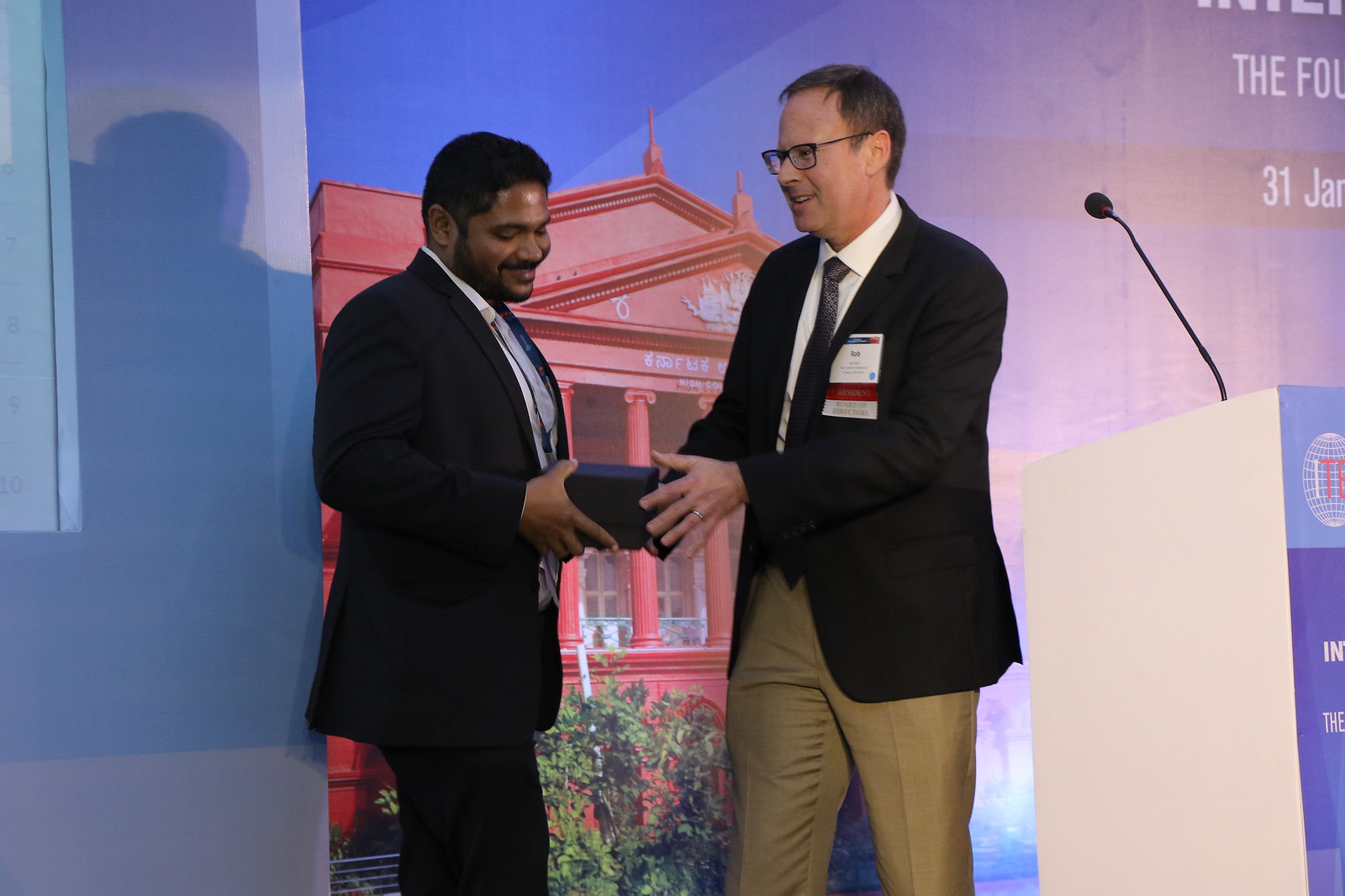This horizontally oriented rectangular image captures a significant moment on a stage between two men, likely during an award ceremony. On the left, a black man with short hair and facial hair, dressed in a black suit with a white shirt and a light purple tie, is smiling while accepting a small black box. He appears to be pleased and intrigued, looking down at the box in his hands. 

The man on the right, who is slightly older with short brown hair and black-framed glasses, is handing over the box. He is also smiling and has a visible name badge identifying him as "Rob," with titles indicating he is the President of the Board of Directors. He is dressed in a black suit jacket, white shirt, and black patterned tie, complemented by khaki pants. His jacket features some kind of identification or lanyard.

In the background, the stage is adorned with a large projector screen depicting an official-looking pink building, which has red pillars and green bushes below it. Flanking either side of the building on the screen are blue and light purple areas, with some partially visible text, including "31 Jan" in the upper right corner. To the far left of the men, a white podium with a blue sign draped over it stands, equipped with a microphone. This detailed composition highlights the ceremonial exchange and the celebratory atmosphere of the moment.